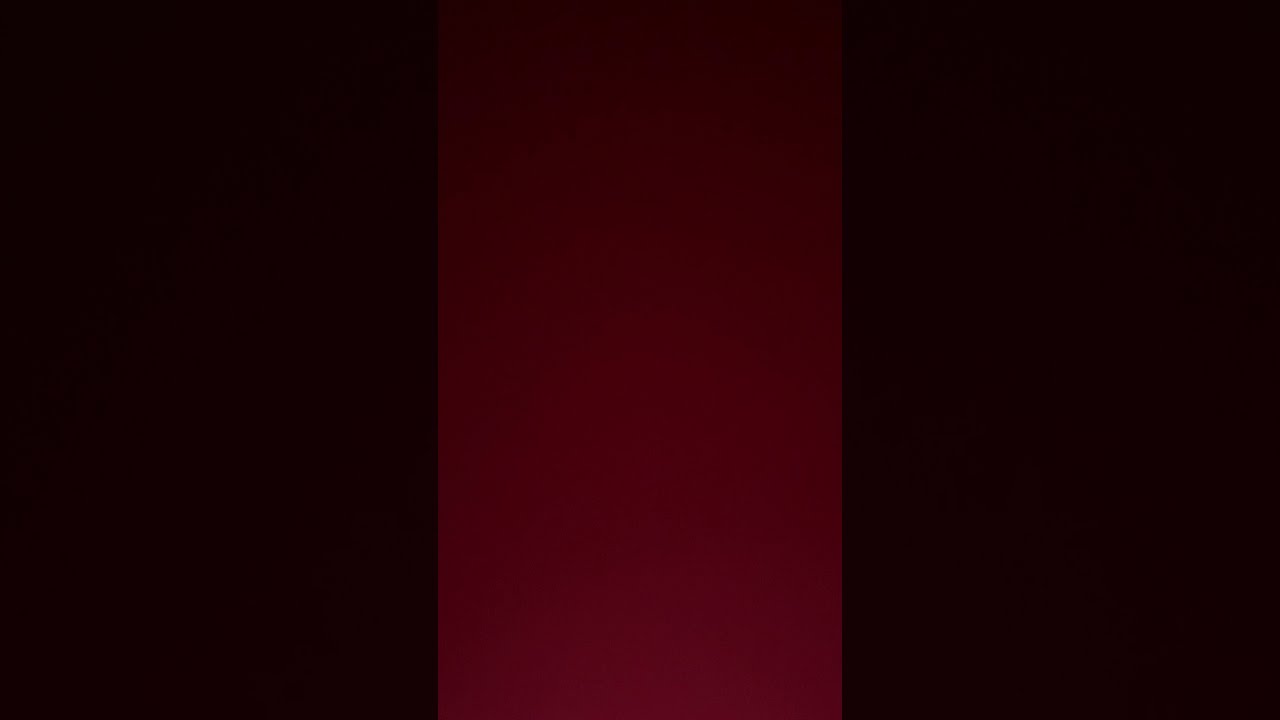The image features a centrally positioned gradient red rectangle, flanked on either side by two nearly identical dark gray-to-black rectangles. The central rectangle boasts a gradient transitioning from a bright, vibrant red at the bottom to a deep, almost black maroon at the top. The coloration is most intense in the bottom right corner and darkens progressively until it becomes completely black in the top left corner. The side rectangles maintain a consistent dark gray hue with subtle maroon undertones. There are no additional elements, images, or text, making the color gradient itself the sole focus of the image.